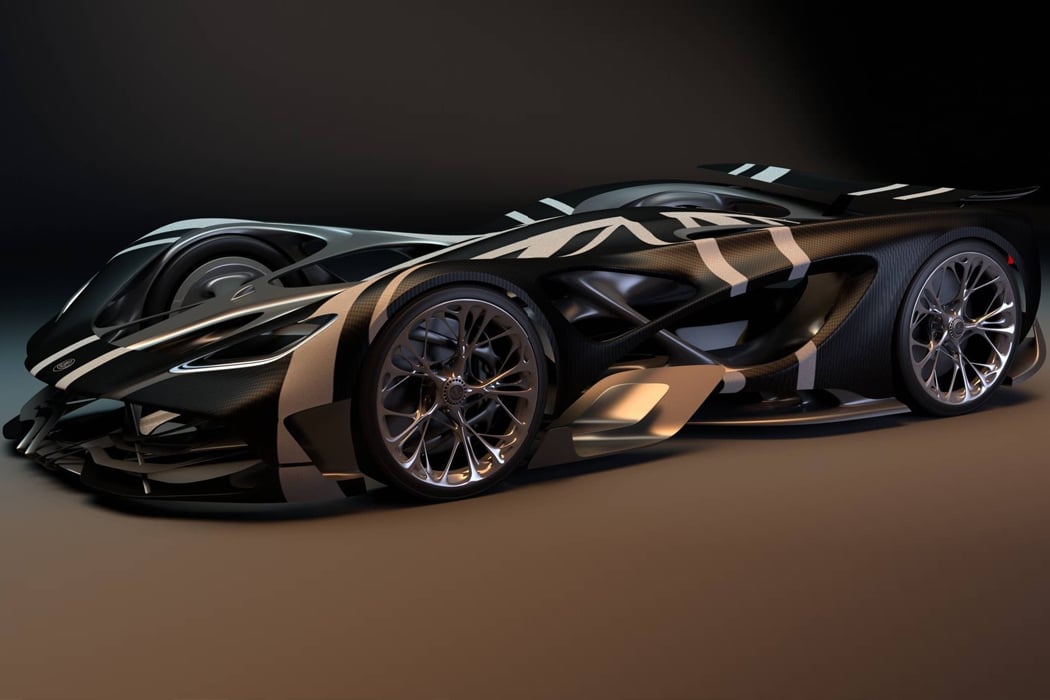The image depicts a high-tech, concept art race car that seems to be AI-generated, as its design appears unconventional and impractical. The vehicle, a sporty black car with intricate white trim, features very large, spider-web-like hubcaps that defy traditional tire attachment logic. The car's design includes sleek edges, and its frame reveals an open section in the rear, allowing visibility of the back wheel, which faces an atypical direction. The car sits extremely low to the ground with minimal clearance, and from the side view, the oversized wheels make the car look squat. The dark background contrasts slightly with the black body, making the silhouette of the vehicle just discernible. Additionally, the car lacks visible doors, suggesting an unconventional entry method, possibly from the top. The design includes gray elements underneath and possibly blue accents, adding to its futuristic aesthetic. The scene is set in a studio room, with minimal lighting, enhancing the car's sleek and enigmatic appearance.